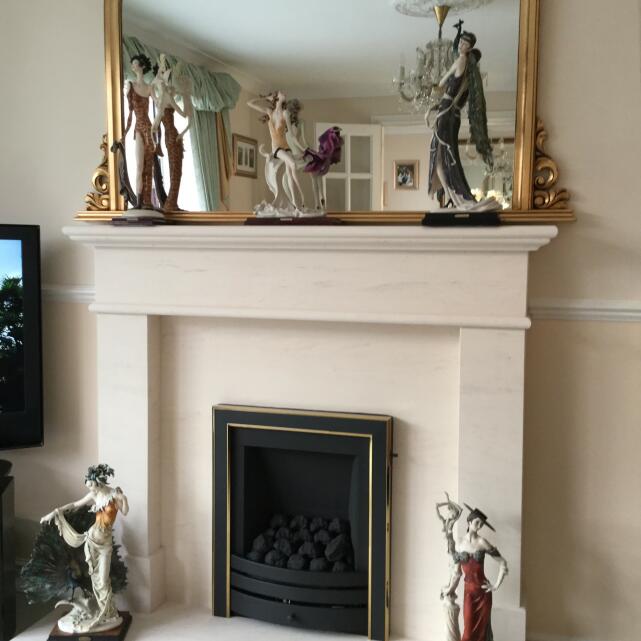The image captures an ornate fireplace showcasing intricate detail and decor. At the center lies a small black and gold fireplace, outlined delicately with gold both inside and out. Within it, uniformly arranged lumps of coal suggest kindling. Flanking the fireplace are two statues of women; the right statue depicts a woman in a red dress with a black hat, while the left features a woman in a long dress situated in front of what appears to be a peacock. Above the fireplace, the white marble mantle holds additional statues of women, evocative of flappers from the 1920s, each posed uniquely. Behind these statues, a large rectangular mirror with a gold frame enhances their display. The room's wall, painted a creamy white, subtly complements the sophisticated setup. On the left edge of the image, part of a flat-screen TV, displaying trees, is visible.